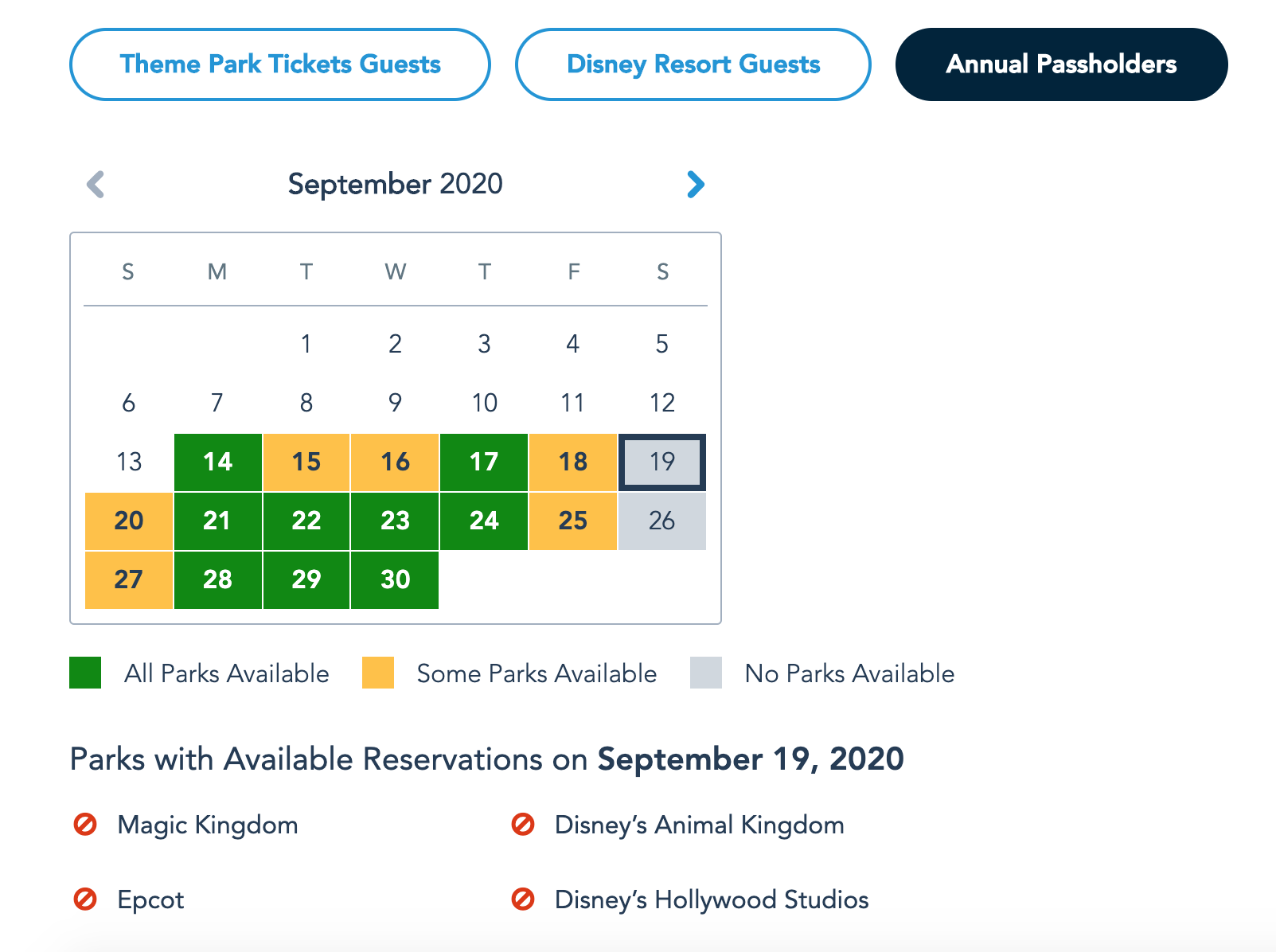The image is a detailed screen capture of a reservation system interface for a Disney park in September 2020. At the top, there are three segmented, oval-shaped tabs: two in blue and one in navy and white. The first blue tab is labeled "Theme Park Tickets Guest," the second blue tab is labeled "Disney Resort Guest," and the navy and white tab reads "Annual Passholders."

Below these tabs is a calendar for the month of September 2020. Navigation arrows are present with a gray arrow pointing left (to go back) and a blue arrow pointing right (to go forward). The days of the week are listed horizontally from Sunday to Saturday. Specific days are color-coded: approximately six days in gold, nine days in green, and two days in gray. 

Underneath the calendar, a color legend indicates the availability of parks: green signifies that all parks are available, yellow indicates that some parks are available, and gray means no parks are available. Additionally, there is a note for "Parks with available reservations on September 19th, 2020," listing Magic Kingdom, Epcot, Disney's Animal Kingdom, and Disney's Hollywood Studios. Each of these parks has a red circle with a slash symbol (indicating no availability) next to them.

The green days on the calendar are the 14th, 17th, 21st, 22nd, 23rd, 24th, 28th, 29th, and 30th of September. The gold days are the 15th, 16th, 18th, 20th, 25th, and 27th. The gray days are the 19th and 26th. 

There are no other notable elements in the image.